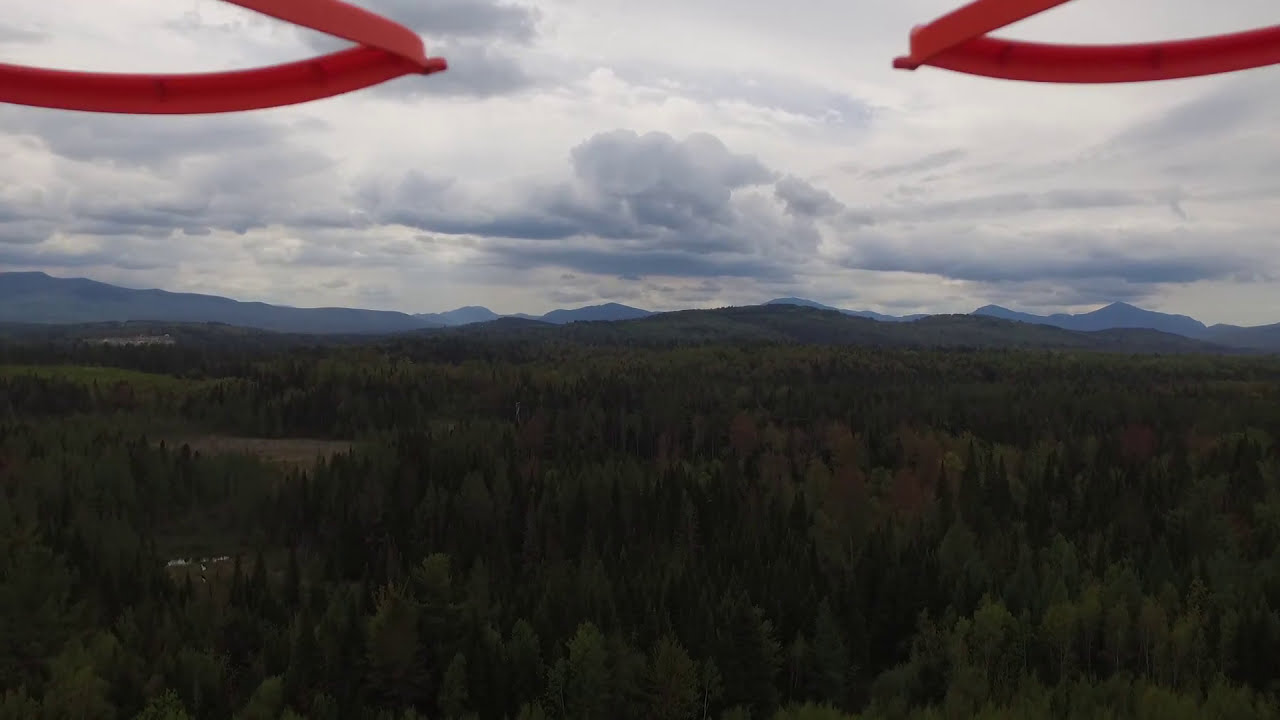This panoramic landscape photograph, likely taken from a high vantage point such as a drone, offers a sweeping view of a dense, green pine forest that stretches into rolling hills and continues all the way to a distant blue mountain range at the horizon. The scene is enveloped in heavy, gray and white rain clouds, blanketing the sky and casting an overcast light upon the terrain. The upper half of the image is dominated by these clouds, contributing to the dark and somber atmosphere. In the top left and right corners of the composition, two mirrored red oval-shaped loops can be seen, possibly part of the drone or the equipment used to capture the image. These elements frame the dense forest below, highlighting the expansive natural beauty of the landscape while adding an intriguing detail to the photograph.